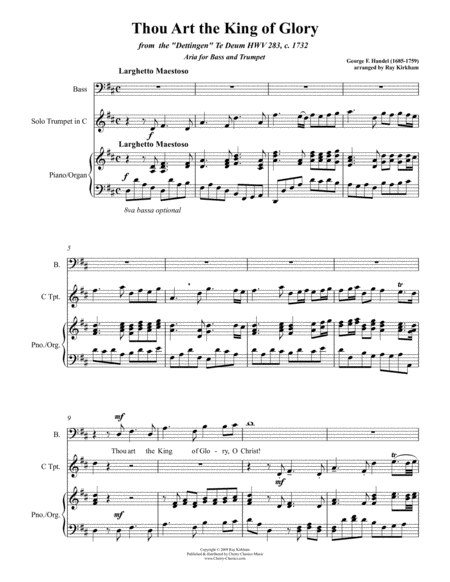This black-and-white sheet music, titled "Thou Art the King of Glory," features bold, dark text at the top. Below it, in smaller print, is written "From the Dettingen," however, the rest of the smaller text is difficult to read. The credited author appears to be "George," possibly George Frideric Handel (1685-1759). The music composition is for bass, solo trumpet in C, and piano organ, organized into three distinct musical lines. The visible lyrical text includes the words, "Thou art the King of Glory, O Christ." The sheet music, believed to be written around 1732, also credits an arranger, though the name isn't clearly distinguishable. This piece is noted for its arrangement and instrumental focus, as inferred from the inclusion of instrumental parts and limited lyrics.